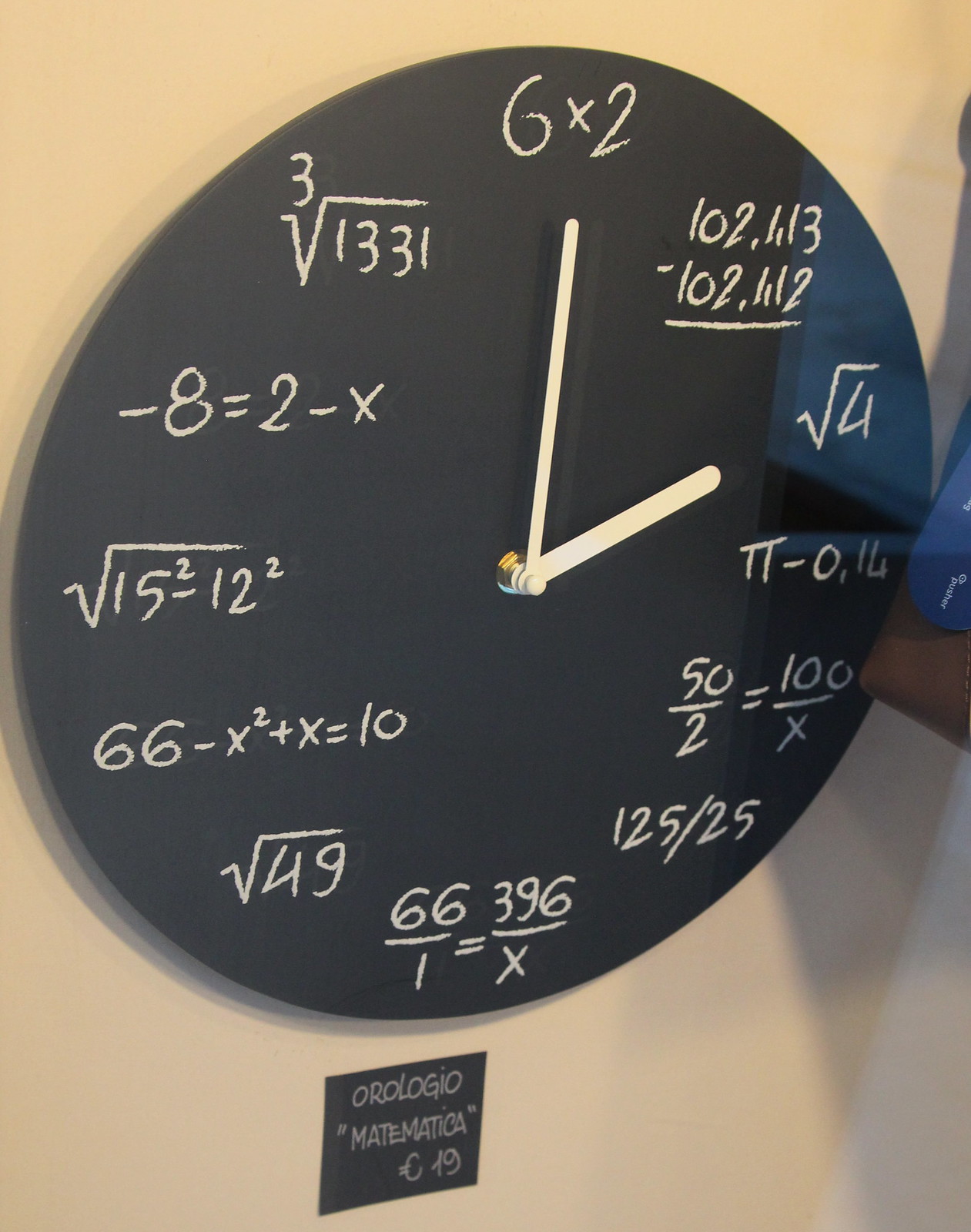This detailed image caption describes a unique wall clock designed with mathematical expressions in place of standard numeral indicators.

---

The image showcases a round, black clock designed to resemble a chalkboard, giving it a quaint and educational appearance. The clock is titled "Matematica," which suggests a mathematical theme. Instead of traditional numbers, each hour mark is represented by a mathematical expression that evaluates to the respective hour. The clock is mounted on a stark white wall, which serves as a clean backdrop to highlight its distinctive design. Below the clock face, there is a label that reads “Orologio Matematica 19,” likely indicating the model or edition of the clock. The pricing is not stated in English, and there’s a notation "C19," which could represent currency or another form of identification.

- At 12 o'clock: \(6 \times 2\)
- At 1 o'clock: \(102,413 - 102,412\)
- At 2 o'clock: \(\sqrt{4}\)
- At 3 o'clock: \(\pi - 0.016\)
- At 4 o'clock: \( \frac{50}{2} = \frac{100}{X} \)
- At 5 o'clock: \( \frac{125}{5} \)
- At 6 o'clock: \( \frac{66}{1} = \frac{396}{X} \)
- At 7 o'clock: \( \sqrt{49} \)
- At 8 o'clock: \(66 - X^2 + X = 10\)
- At 9 o'clock: \(\sqrt{15^2 - 12^2}\)
- At 10 o'clock: \(-8 = 2 - X\)
- At 11 o'clock: \( 3 \times \sqrt{1,331} \)

This creative and educational timepiece would be perfect for math enthusiasts or anyone looking to bring a touch of intellectual charm to their space.